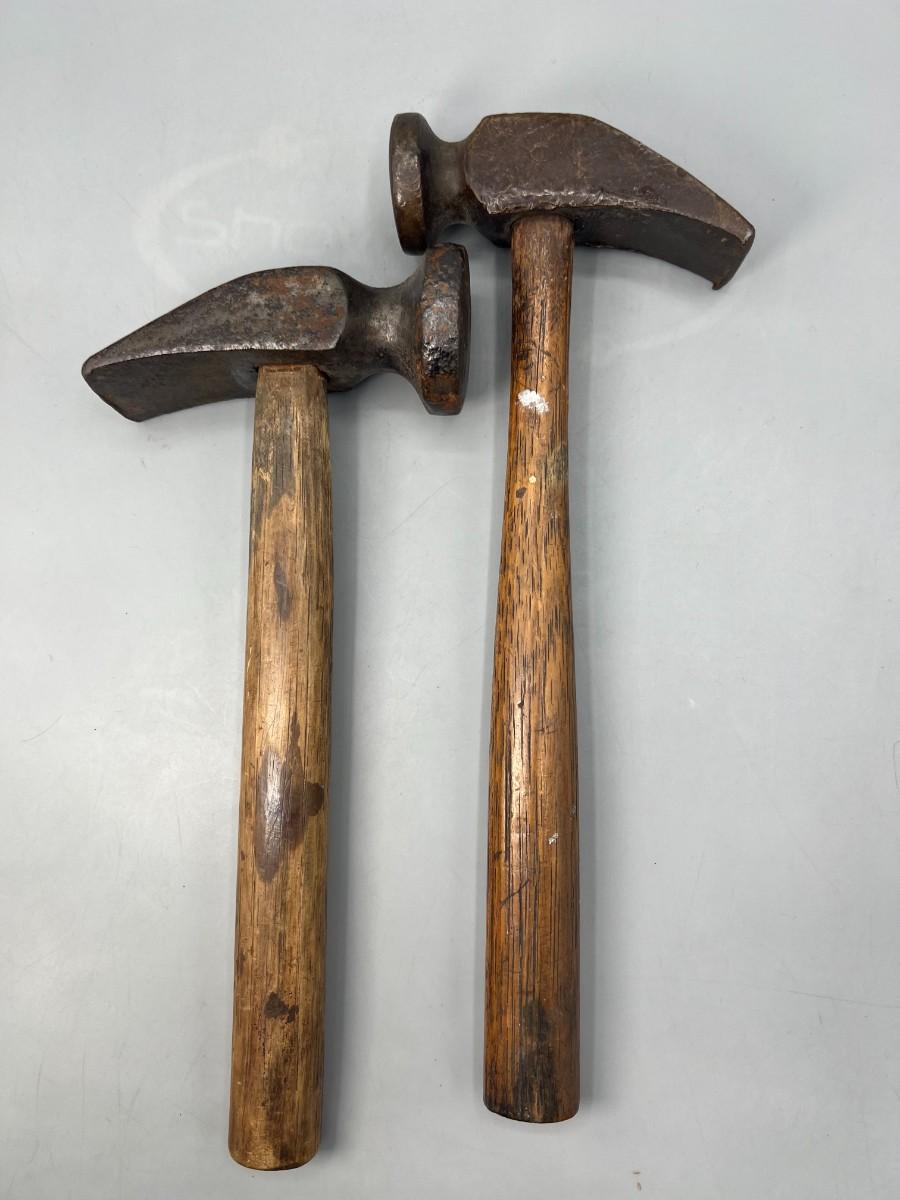This top-down photograph features two antique wooden-handled hammers resting on a light gray surface, possibly a piece of gray paper or cloth with a faint logo or watermark visible, possibly forming the letters 'S-H-O-W'. The hammers are positioned almost parallel to each other, with the right-hand hammer slightly elevated above the left, causing their heads to overlap slightly. Both hammerheads are dark gray metal, exhibiting various wear marks and slight rust, more so on the left hammer. Unlike modern hammers, their claw backs are wedge-shaped rather than the typical V-shaped notch meant for nail pulling. The wooden handles appear aged and weathered, with visible white paint splatters and varying shades of dark and light spots from extended use. The handles give off a handcrafted look, suggesting they might have been locally forged or produced rather than mass-produced. The overall image composition, with shadows indicating a top light source, emphasizes the details and aged characteristics of these tools.